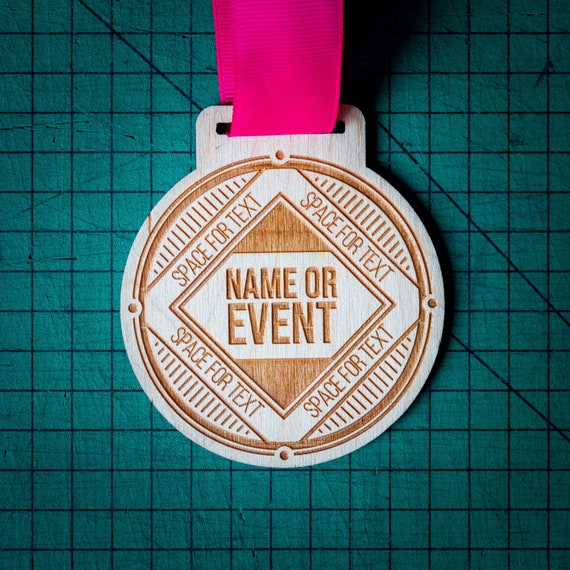This image is a detailed close-up of a medal, which appears to be designed as an award template. The background is a dark green paper divided into small squares by black lines, creating a grid-like pattern. In the top middle, a pink ribbon or strap descends through a small slit in the top of the medal, with a portion of the ribbon also visible to the left of the slit. 

The medal itself is constructed from a light-colored material, possibly wood or metal, with specific sections inlaid with a darker brown color. The top of the medal features a white section with a slit for the ribbon. Below this, there's a gold-outlined circle in the center of the medal. Within this circle is a square rotated to resemble a diamond, outlined in brown. Inside this diamond-shaped square is another smaller square, also rotated, which contains the placeholder text "name or event" in brown.

The outer diamond shape has space designated for text on all four sides—top left, top right, bottom left, and bottom right—each marked "space for text." The areas of the circle not occupied by the diamond display small brown lines extending from the edges of the diamond to the circle's edge, filling the space.

The overall composition of the medal, with its intricate design intended for customization, lies on the green grid-patterned background, emphasizing the layout and decorative elements of the award.